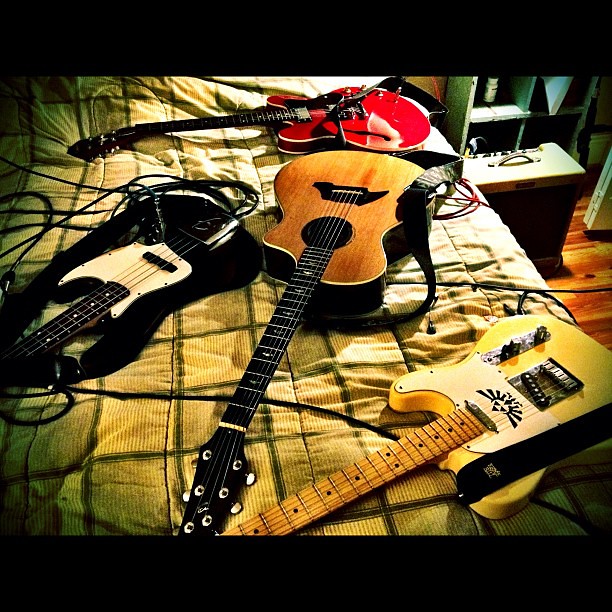The photograph showcases a varied collection of four guitars arranged haphazardly on a bed with a yellow and brown crisscross-pattern comforter. Anchoring the display is a vibrant red electric guitar with a black neck, appearing horizontally at the top. Below it lies a blonde-faced acoustic guitar with a contrasting black neck. Adjacent to the acoustic guitar is a black and white electric guitar. Positioned prominently in the foreground is a distinctive yellow electric guitar, featuring the Zelda Triforce symbol between its pickups. To the right, the wooden floor is visible, along with a small amplifier on the floor and a bookcase or drawer with what appears to be a jar or bottle inside.